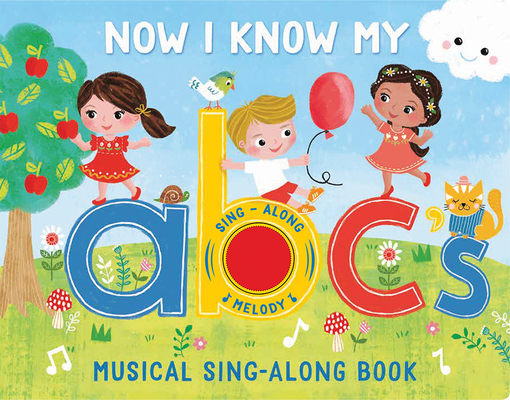The cover of the children's musical sing-along book titled "Now I Know My ABCs" bursts with vibrant, playful detailing in a charming park-like scene. The backdrop features a lush green lawn with yellow highlights, a sturdy brown tree adorned with four red apples, and a blue and white sky. At the upper right corner, a cheerful white cloud with rosy cheeks and a blue smile beams down, with its words reading, "Now I Know My ABCs, music sing-along book."

Central to the illustration are the large, colorful letters A, B, C, and S arranged on the grass. The blue 'A' supports a girl in a red dress, stretching upwards as if reaching for one of the apples. Adjacent, a boy with blonde hair, dressed in a white shirt and yellow shorts, sits comfortably on the yellow 'B.' He holds a bright red balloon while a colorful bird with a green head, yellow beak, and white body perches beside him. The boy's orange sneakers add a splash of yet more color.

Next to them, on the C, stands another girl with brown hair and a brown complexion. She wears a pinkish-orange dress and appears to be dancing. Her setting is brightened by a daisy with white petals and a blue center positioned behind the C. Between the B and C, two mushrooms with red caps and white spots add a whimsical touch.

Completing the scene, an orange cat with white stripes and a blue apron-type clothing sits serenely on the letter 'S,' while another daisy with a red center and a green stalk and a mushroom with spotting nearby add to the delight. The ground features varied greens and a hint of yellow, tying together this lively, enchanting cover designed to captivate and invite young readers into the musical journey of learning ABCs.